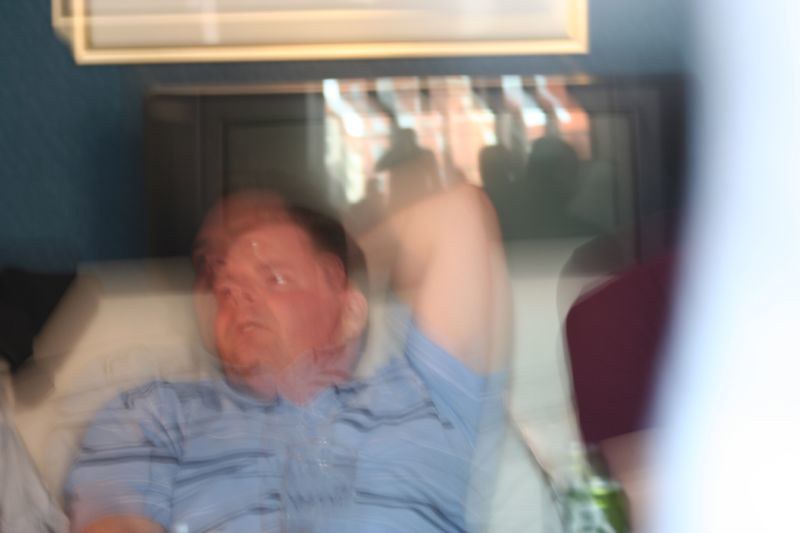In this very blurry, possibly double-exposed photograph, a white man with short dark hair is laying on an adjustable hospital bed or a similar type of bed where the back can be raised. He is leaning slightly upwards with his left arm bent behind his head, looking diagonally to his right. He is wearing a short-sleeved polo shirt with light blue and dark blue horizontal stripes. His right arm is not clearly visible in the image. The man is situated on a white surface, likely a pillow or part of the bed. A green and silver can is noticeable on a table near the bottom right-hand side of the image. There appears to be a reflection, possibly in a mirror or through a glass window behind him, showing multiple people either standing or sitting and facing him. A black TV, which is not in use, is also discernible in the background along with other indistinct shapes and colors.